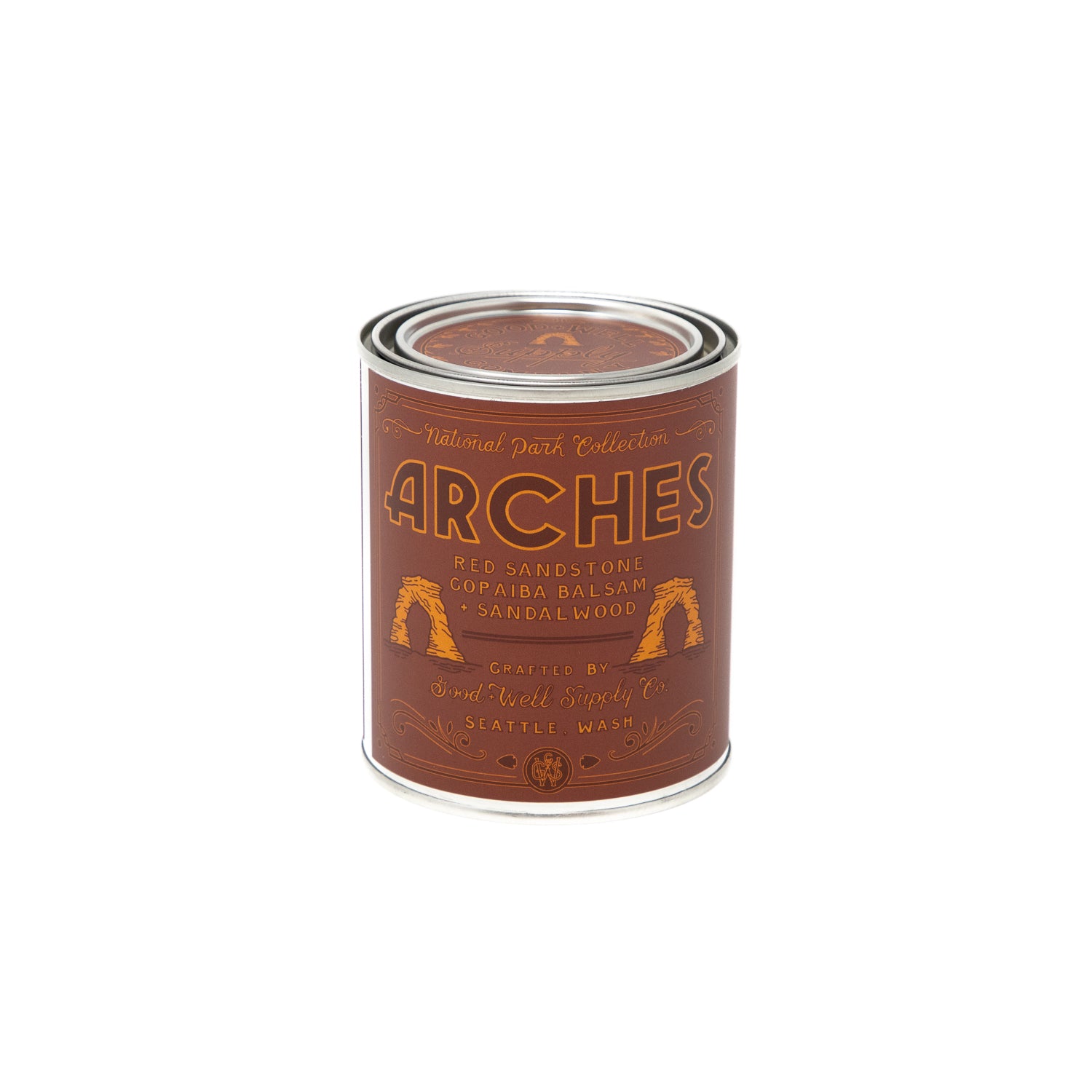This image features a sealed metal can with a removable and replaceable lid. The can is adorned with a rustic brown paper label set against a white backdrop. The label prominently displays "National Park Collection" in script at the top, followed by "Arches" in dark brown text, trimmed in golden orange. Below this, detailed in slightly smaller text, are the words "Red Sandstone, Copaiba Balsam, Sandalwood." On either side of the word "Sandalwood," there are artistic drawings of natural arches. The can is labeled as a product crafted by Goodwell Supply Company, Seattle, Washington. The item is an Arches National Park candle, evoking the scents and essence of the park with notes of Red Sandstone, Copaiba Balsam, and Sandalwood.